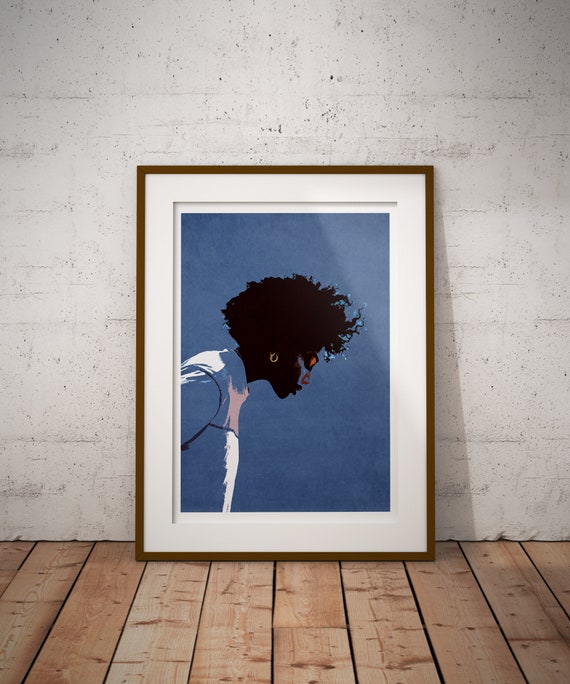A framed painting is positioned against a white brick wall on light brown wooden plank floors. The frame itself is dark brown with a white bevel mat inside. The artwork features a deep navy blue background with a prominent profile of a woman facing downward from the left side. Her hair is a poofy, fluffy, black silhouette, contrasting against the blue. The woman's eyes are closed, adorned with orange and reddish eyeshadow. Her nose has red highlights and a hint of blue. She is wearing small gold hoop earrings and a white-grey shirt. Only the upper portion of her body is visible, extending just below the chest. The painting, which exudes a mix of mystery and serenity, is centered within the frame.